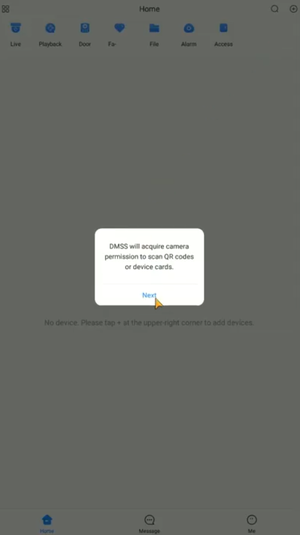The image is a vertically oriented rectangular screen. Dominating the central part of the screen is a prominent pop-up window. The pop-up, a clean white box, features blue text that reads, "DMSS will acquire camera permission to scan QR codes or device cards." At the bottom of this pop-up is a blue "Next" button, highlighted further by a small orange arrow pointing directly at it.

The background of the screen is obscured by a dark gray overlay, making it challenging to discern the details. However, faint outlines of some background elements are visible. Across the top of the screen are approximately seven blue icons, among which the word "Home" is legible. Additionally, there are a few indistinct icons located at the bottom of the screen. The overall ambiance of the image is dim due to the shaded overlay, focusing attention on the pop-up window.